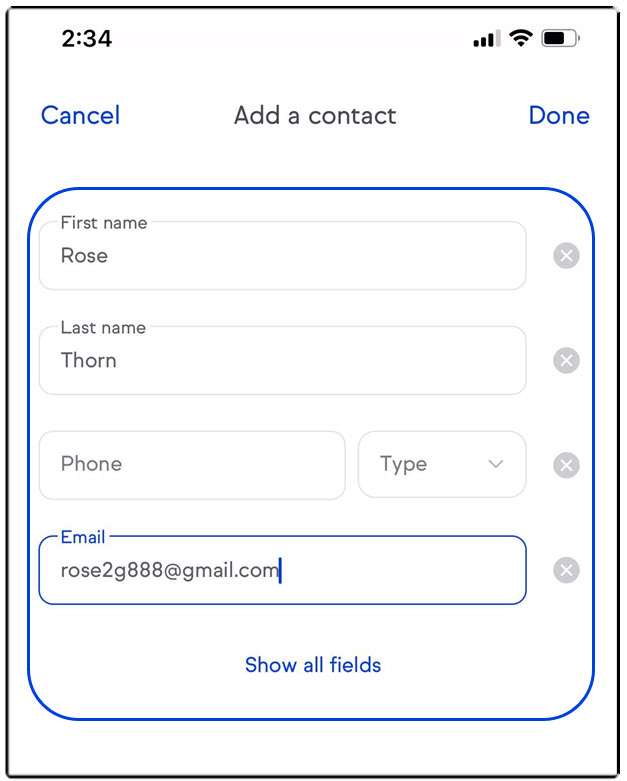This screenshot captures a smartphone interface displaying the contact addition screen. The image, centered and vertically elongated, shows the time as 2:34 at the top left corner, while the top right corner indicates three bars of signal strength, active WiFi, and a half-full battery icon. Just below this status bar, "Cancel" appears in blue text on the left, "Add a Contact" is centered in black text, and "Done" is in blue text on the right.

The main section underneath features a blue-outlined square with rounded corners, designated for entering contact details. Input fields within this area include "First Name" filled as Rose, "Last Name" filled as Thorn, an unspecific section for a phone number, another for selecting the type, and an "Email" category populated with rose2g888@gmail.com. Towards the bottom center of this screen, the option to "Show All Fields" is presented in blue text.